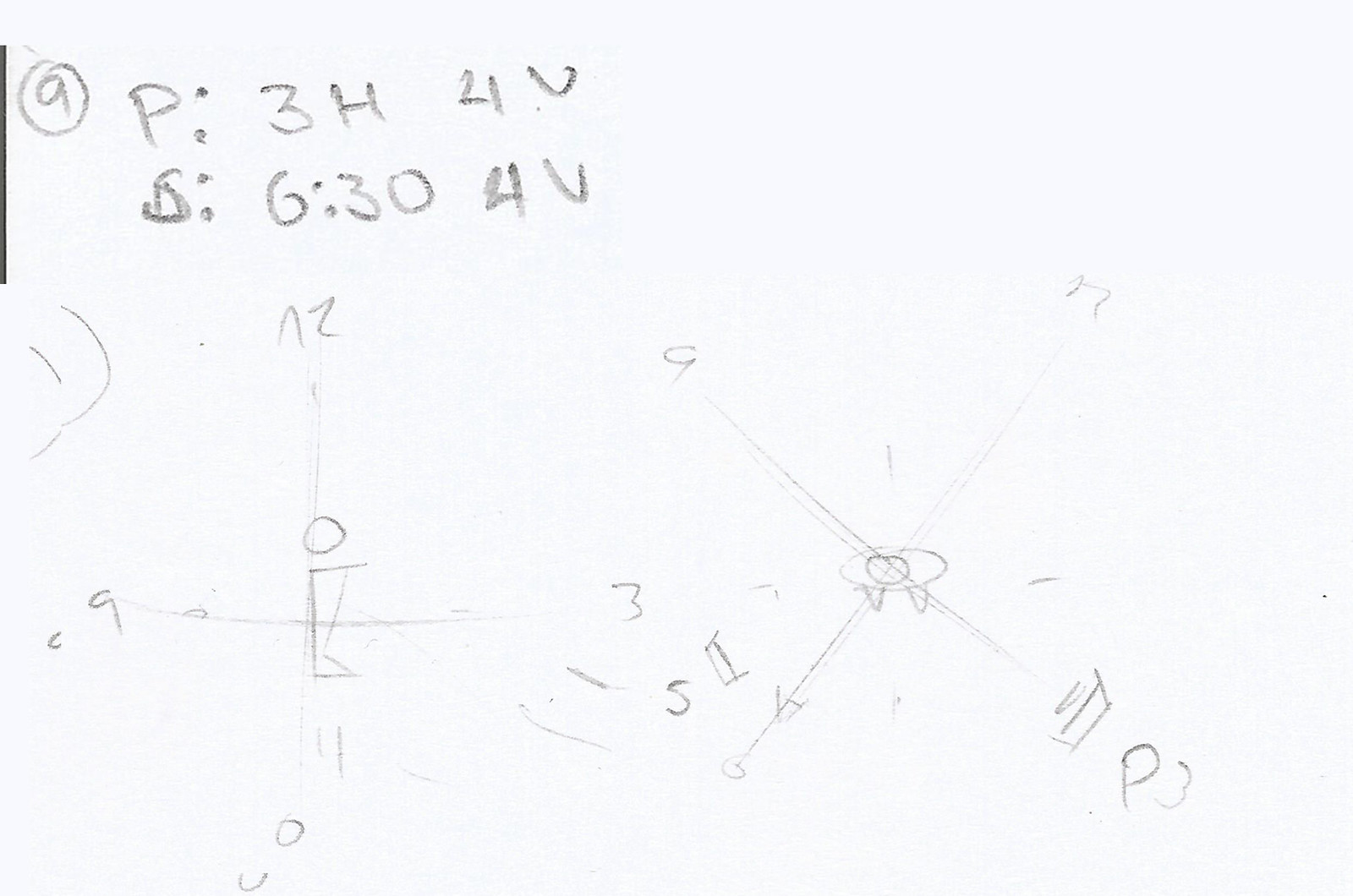The image displays a scanned piece of paper featuring hand-drawn elements and annotations. In the upper left-hand corner, the number "9" is prominently circled, indicating it as the answer to question number nine. Below this, there are cryptic alphanumeric sequences and symbols, likely serving as part of a puzzle or riddle. The first line reads "P:: 3H4V," and beneath it, another line that resembles "D or B : 634V."

Further down, there are two distinct drawings. On the left, a vertical line intersects with a horizontal one, creating a cross. At this intersection, there is a circle and an additional geometric shape resembling two triangles conjoined at their points. On the right side, an "X" shape is formed by intersecting lines. At the center of this "X," a smaller circle is surrounded by a larger one, and attached to the bottom of the larger circle are two triangular shapes forming a "V." This composition suggests a structured but abstract conceptual drawing, possibly part of a larger puzzle or diagram.